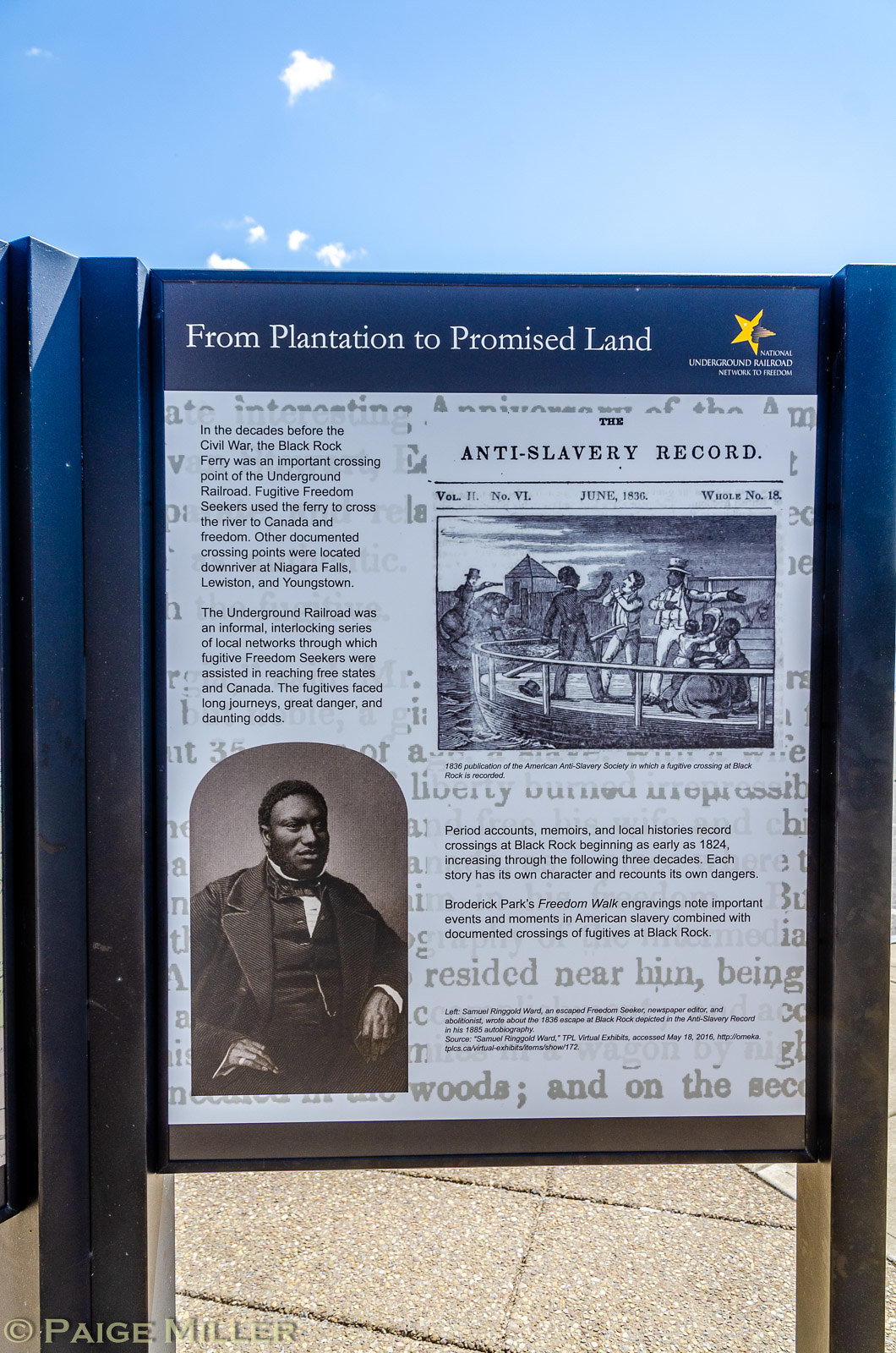The image is a photograph taken outside on a partly cloudy day, capturing an informational plaque typical of those found at historical sites. The plaque, mounted on black metal posts, features a blue header with white text that reads, "From Plantation to Promised Land," and includes a yellow star in the corner underneath the title. The plaque is primarily white with tan words scattered across the background, featuring prominent terms like "liberty," "reside near him," "being," "woods," and "anti-slavery record."

On the left side of the plaque, there is an arched, framed, sepia-toned photograph of a well-dressed black gentleman. He is seated, wearing a fine suit, a scarf around his neck, and a buttoned vest. To the top right, there is a black-and-white sketch depicting people being transported by boat, likely referencing the forced migration of African Americans. The plaque includes three to four paragraphs of explanatory text detailing the significance and history of the gentleman featured in the photograph.